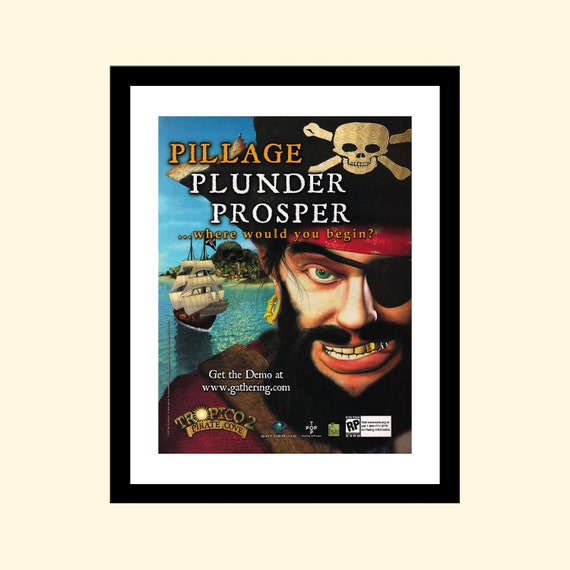The image is a color photograph of a framed poster, prominently displayed on a light yellow or white wall. The black frame features a white mat that enhances the vibrant scene within. At the center of the artwork is a highly detailed, realistic rendering of a pirate's face. He wears a traditional black pirate hat adorned with a skull and crossbones, and a red bandana peeks from underneath. One eye is strikingly green, while the other is covered by a classic eye patch. His dark black beard includes a full goatee, and his expression is menacing, with several golden teeth glittering through his snarled visage. 

Behind the pirate, the background features a distant pirate ship sailing on the ocean, flanked by a lush grove of trees and an island. The poster includes the prominent text: "Pillage, Plunder, Prosper. Where would you begin? Get the demo at www.gathering.com," suggesting it is an advertisement for the video game Tropico 2, Pirate Cove. The overall composition of the poster effectively captures the adventurous and piratical theme of the game.